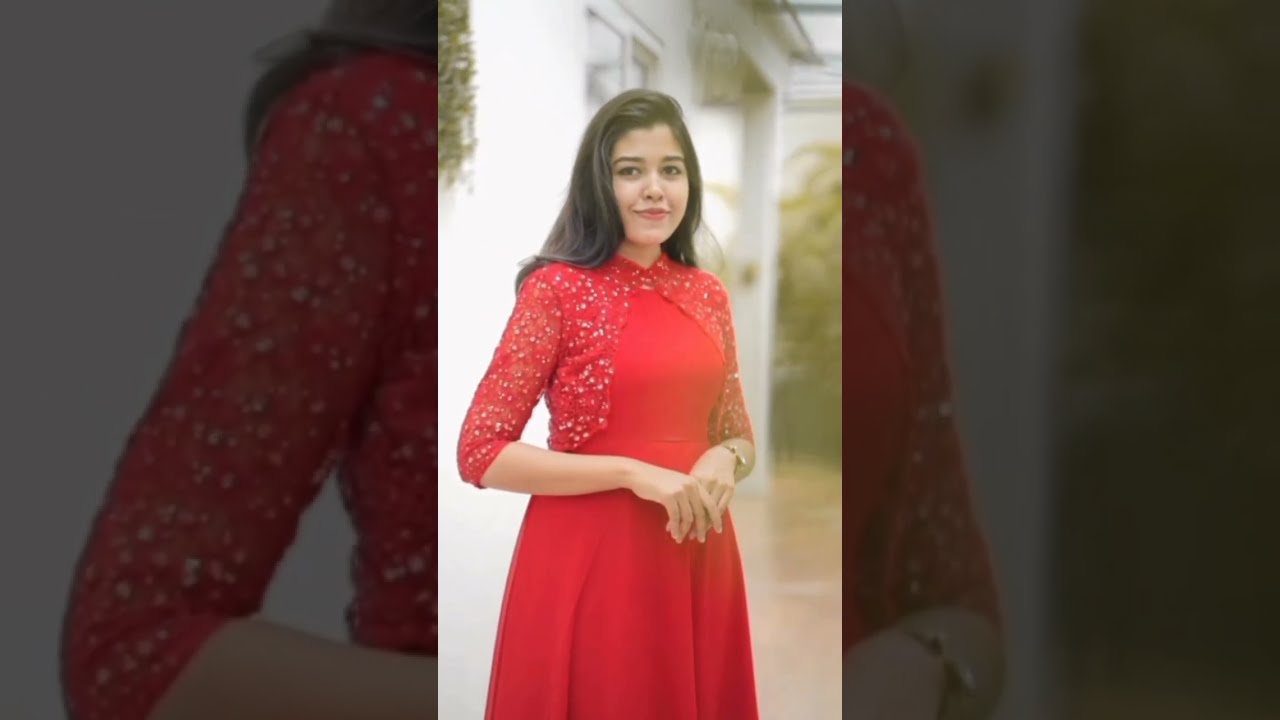The image is divided into three vertical sections. The middle section features a photograph of a young lady standing and facing the viewer at a slight angle. She is wearing a long red dress with a matching bolero jacket adorned with shiny studs. Her long brown hair is swept over to the right side, and she is smiling with her lips closed, revealing pink lips and brown eyebrows. Her hands are joined together in front of her body, with her fingers pointing downward, and she is wearing a gold watch on her left wrist. In the background, there is a white house with a visible window and an overhang. To the upper left of the image, some shrubbery can be seen, although the background is slightly out of focus. The first and third vertical sections are slightly darkened close-ups of the central image, creating a wide, dull, and grayed-out border around the young lady in her vibrant red outfit.